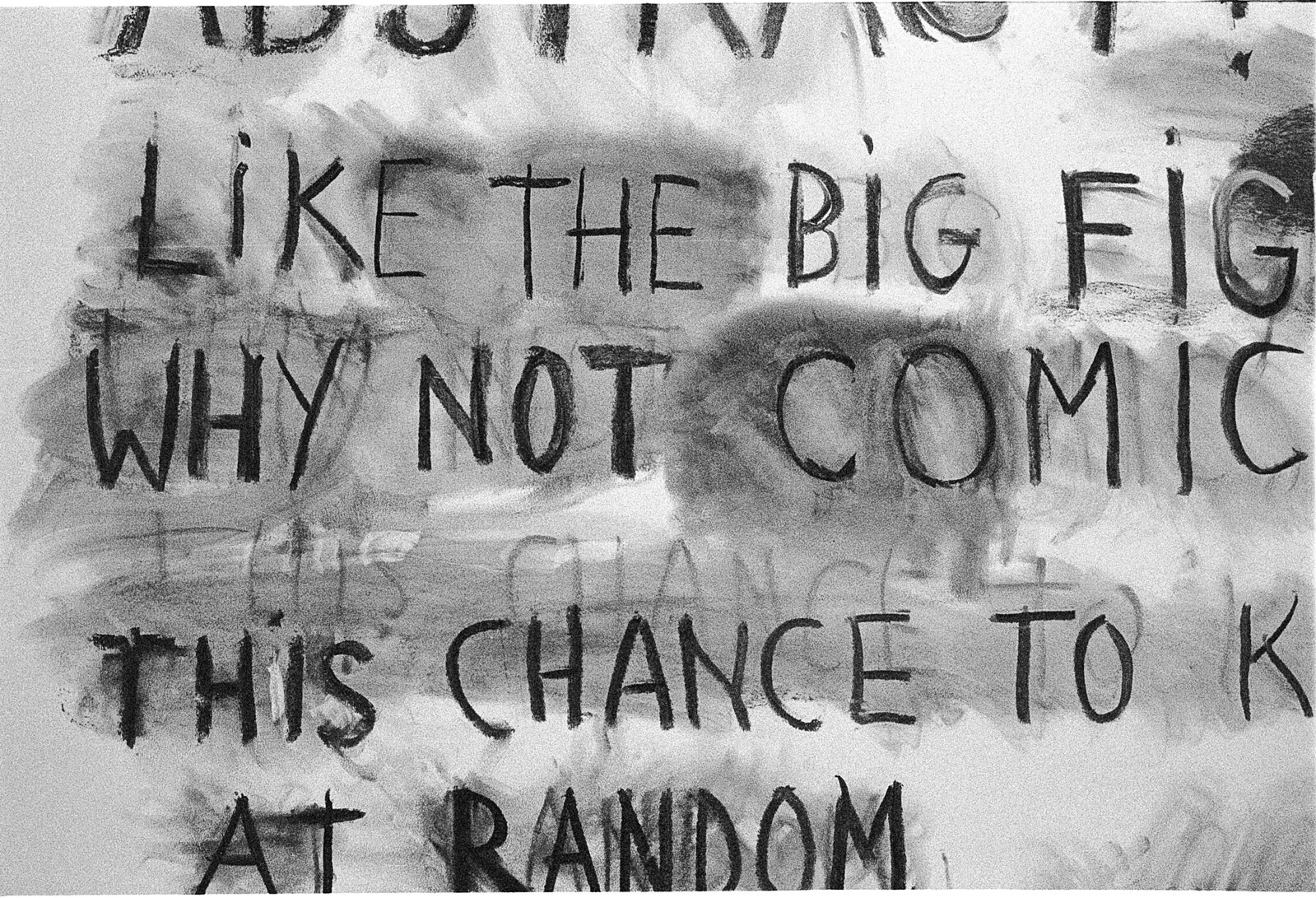The image depicts a haunting, horror-themed sign with black text inscribed on a light gray background marred by dark, hand-smeared smudges, resembling the effect of repeatedly erased charcoal. At the top, some text is partially cut off and unreadable. Below it, in bold black print with a shadowy, repeated echo effect, the words "like the big fig" appear. Following this, the fragmented and layered phrases "why not comic," "this chance to K," and "at random" are visible. The entire composition of the text is disjointed, contributing to an eerie and disordered aesthetic, enhanced by the overlapping and incomplete sentences amidst blurred and smudged gray tones.